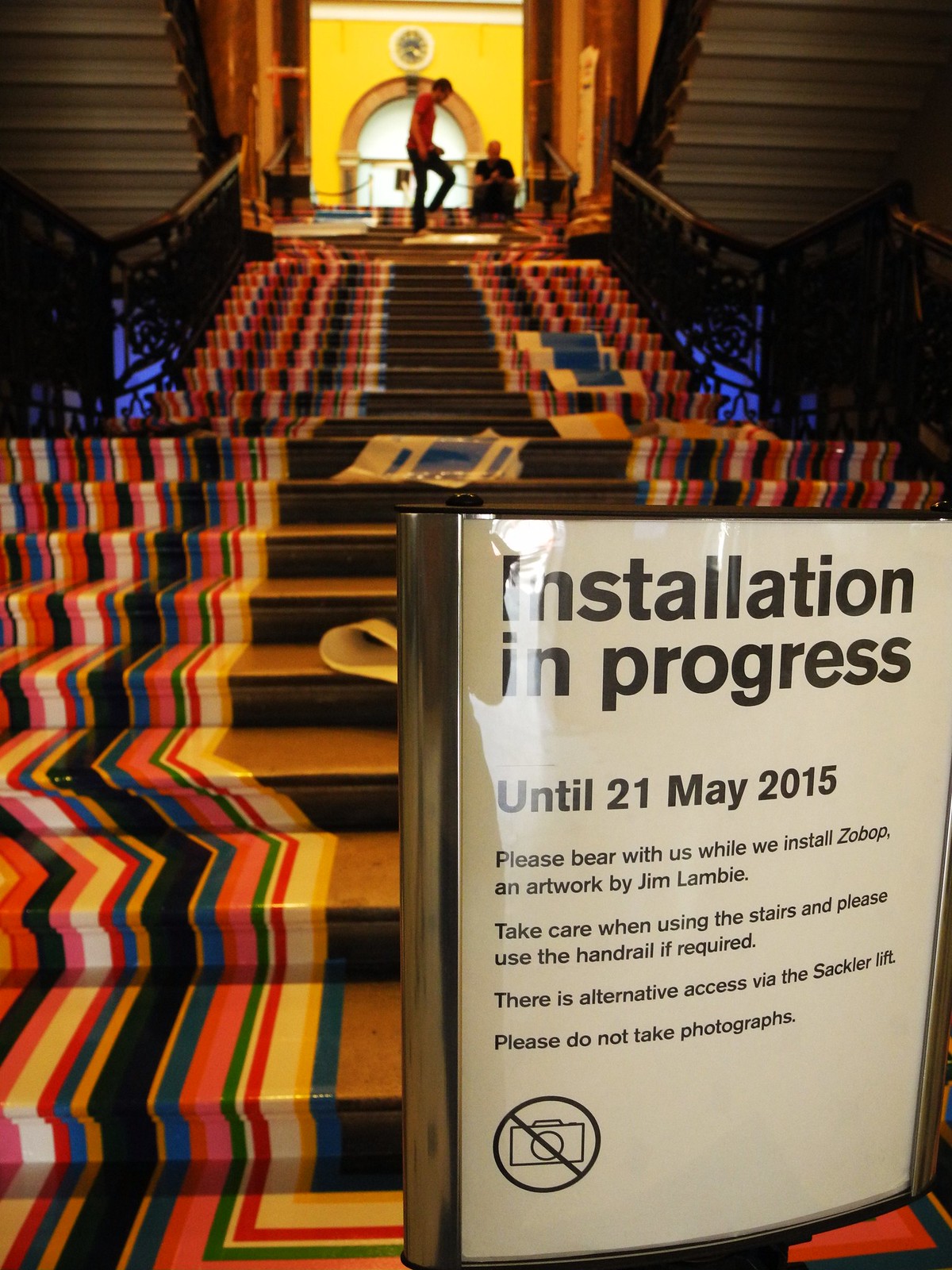The image features a wide, multi-level set of stairs located in what appears to be an elegant building or museum. The most eye-catching aspect is the striking rainbow-like pattern of vivid colors—blue, yellow, white, red, green, pink, orange, black—that adorn the left and right sides of the stairs, while the center remains a solid black. There are numerous steps, possibly 30 to 40, extending upward to the next level, where additional flight of stairs leads in opposite directions on both sides. 

At the bottom right of the image, there is a large, laminated white sign with a metal border, prominently displaying black text: "Installation in progress until 21 May 2015. Please bear with us while we install ZoBop, an artwork by Jim Lambie. Take care when using the stairs and please use the handrail if required. There is alternative access via the Sackler Lift. Please do not take photographs," accompanied by a crossed-out camera icon. In the distance, a few individuals appear to be installing additional signs at the top of the staircase.